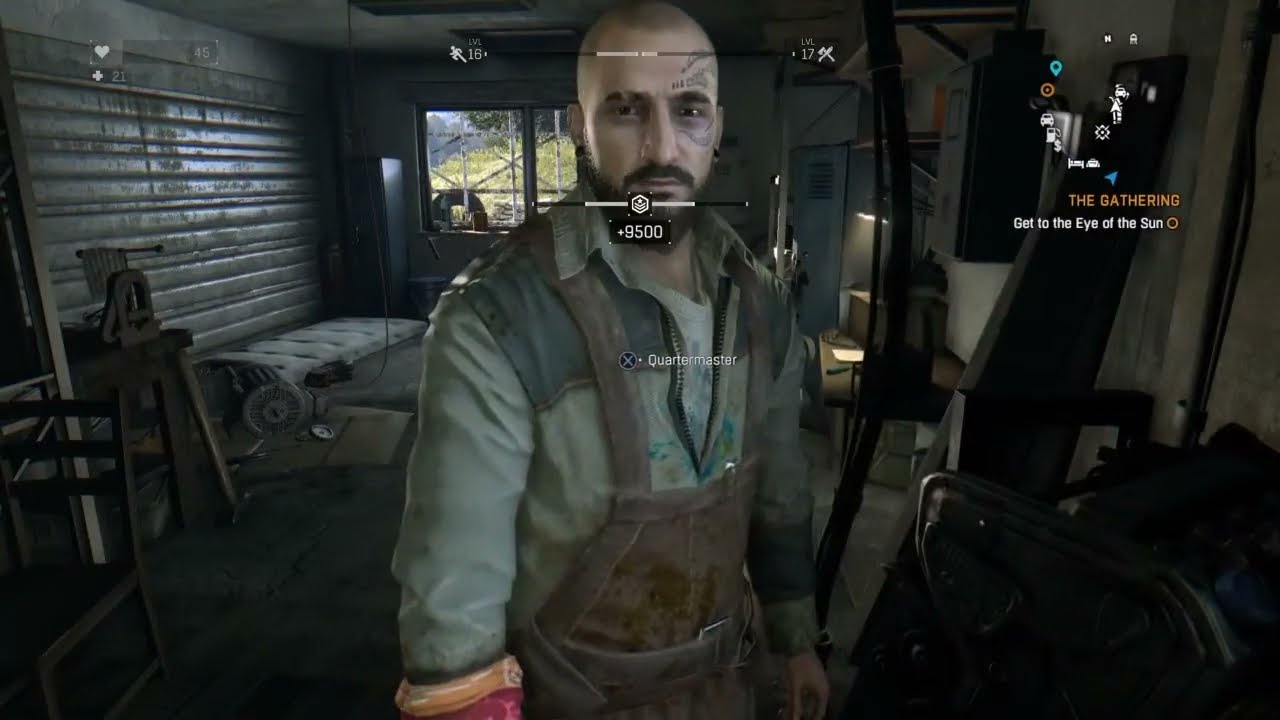The image is a still frame from a video game showing a character in a worn, dilapidated room that resembles a storage unit or shed. The central figure is a white man with a bald head, a dark beard, and a mustache. He has distinctive black wave tattoos around his right eye and wears dirty brown overalls over a light green, zippered, collared jacket with a white undershirt beneath. Text overlays the image, with "Quartermaster" and "+9500" displayed across his chest, along with an X button symbol. The room's background features various items: an old, white mattress against a metal rolling door, industrial equipment, a workbench, lockers, and a chair. A window reveals green grass outside, enhancing the dystopian feel. In the top right corner, there is a map with icons forming a circle and the text "The Gathering: Get to the Eye of the Sun." The top center of the image displays a progress bar indicating a level upgrade from 15 to 17.